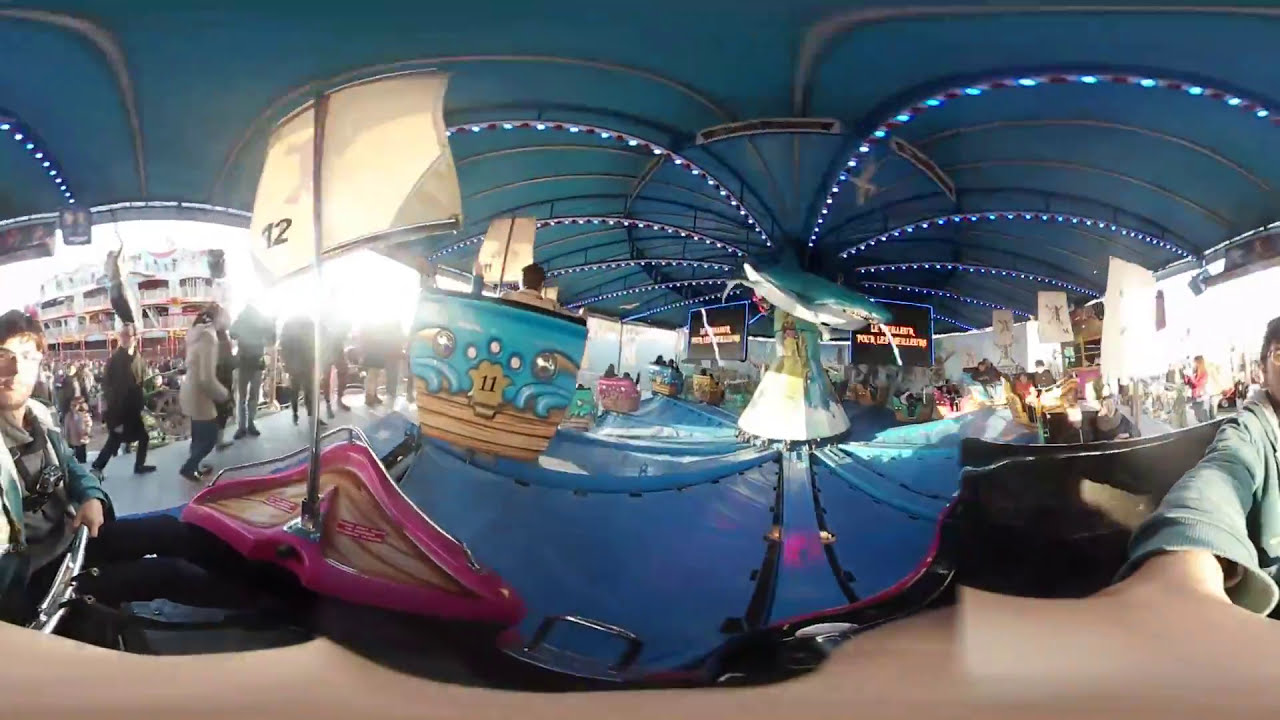The image captures an indoor play area or arcade, characterized by a dominant blue theme. The light blue ceiling features multiple strips of blue LED lights radiating from the center, creating a playful and vibrant atmosphere. In the middle of the image, a central pillar showcases a large 3D shark statue, painted in blue and white, as if it is emerging from both the pillar and the ceiling. The pillar itself is adorned with various sea life illustrations, enhancing the underwater motif.

Below, the floor is also blue and houses several black rods extending from the pillar. Each rod supports a boat-shaped vehicle, which are colorfully painted in nautical themes and equipped with small flags or sails on silver poles, each with a number on it. In the forefront, a man wearing glasses operates the camera. To the left, a person sits in a boat secured by a silver metal bar across their lap, with a pink triangular panel and a pole in front of them. Another person on the left side of the image is leaning forward, their hand stretched out. The scene is bustling with people walking around, engrossed in the lively environment typical of an arcade or an indoor carnival ride area.